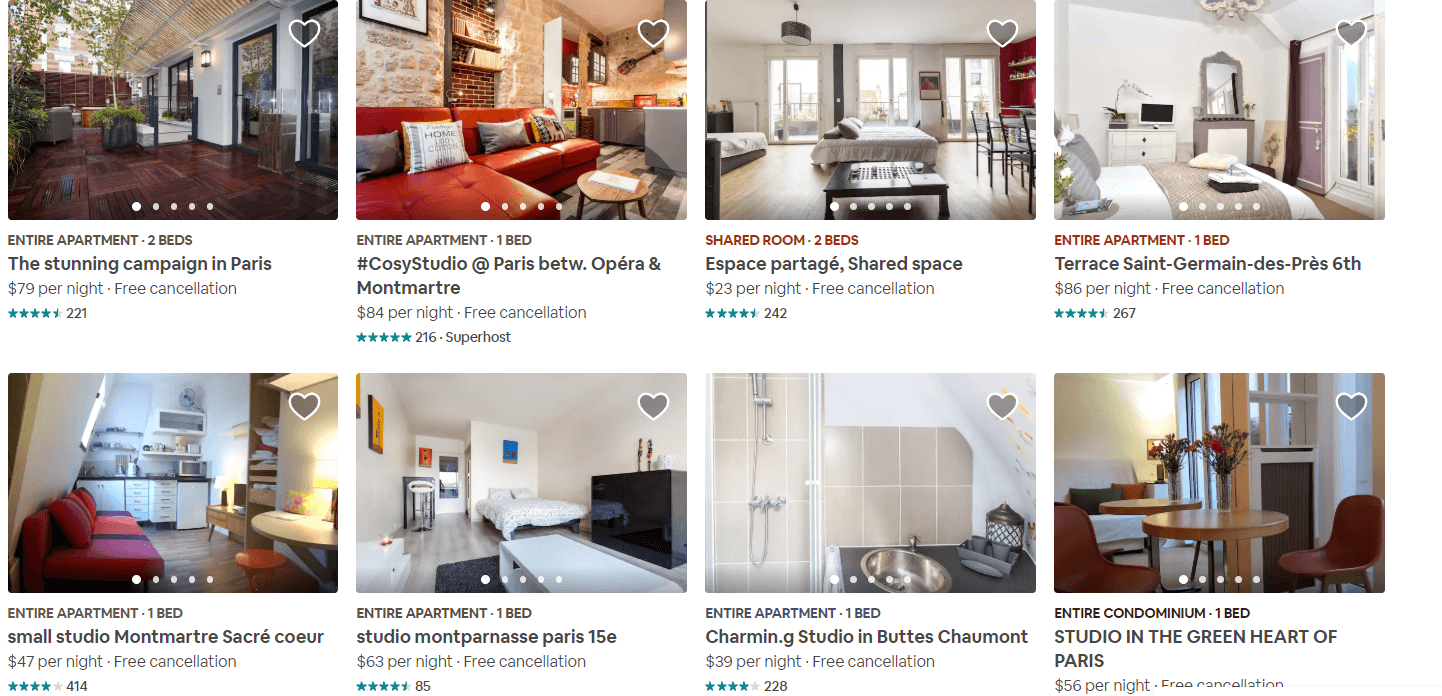The image depicts a web page, likely for a rental service akin to Airbnb, showcasing eight different rental options arranged in two rows, each featuring four properties. Every listing includes a photograph and key details about the rental. In the top right corner of each image, there is a white-outlined heart icon, suggesting users can favorite the listing.

Highlighting a specific example, the first rental is an entire apartment in Paris, featuring two beds and described as a "stunning campaign." It is priced at $79 per night and includes free cancellation. This free cancellation policy is consistent across all listings. 

Each rental item mentions the nightly rate, the type of accommodation offered (e.g., entire apartment, shared room, bedroom), and a star rating at the bottom to indicate user satisfaction. Among these options, the most economical choice is a shared room with two beds, available for just $23 per night.